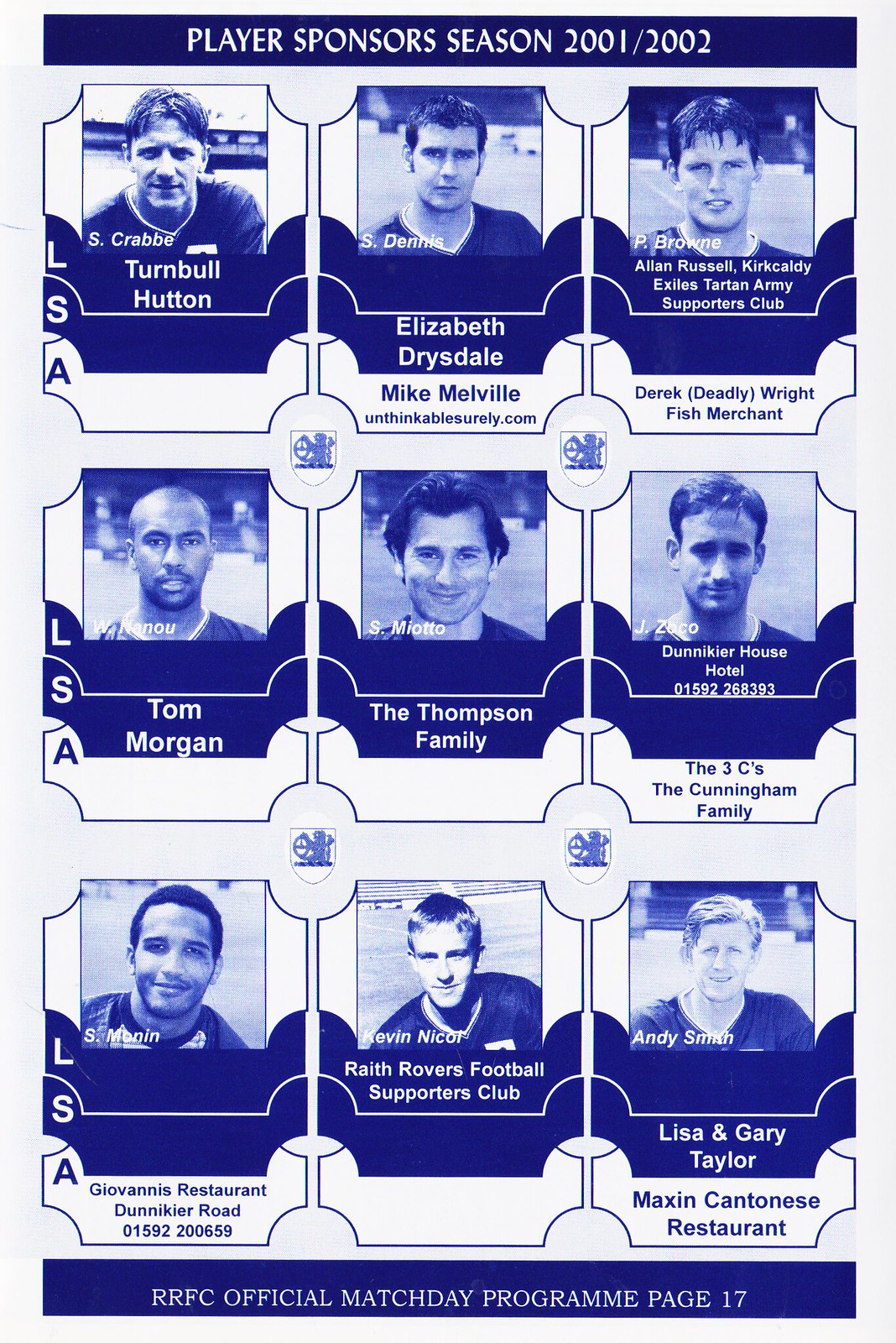This detailed page from the RRFC Official Match Day Program for the 2001-2002 season, found on page 17, features nine black and white photos arranged in three rows of three, all tinted with a blue hue. Each player's image is prominently displayed with their name directly on the photo. Above the image section, a blue-bordered heading reads "Player Sponsors Season 2001-2002." The top left image showcases Turnbull Hutton, followed by S. Dennis in the middle row, whose photo is accompanied by sponsors Elizabeth Drysdale and Mike Melville beneath it. Other player photos display similar layouts, with one or two sponsors listed below each, such as S. Crabb and other identified players. The sponsors include notable names like Derek Deadly-Wright, Fish Merchant, Tom Morgan, The Thompson Family, Jenneker House Hotel, Giovanni's Restaurant, and Faith Rover's Football Supporters Club, among others. The consistency in the blue and white color palette enhances the visual unity of the program page, underscoring the connection between the players and their sponsors.